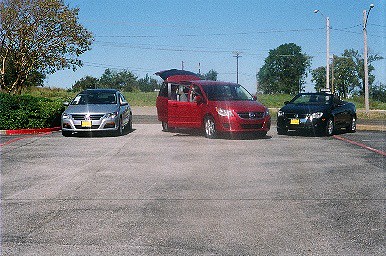This photograph, likely taken with an old digital or 35mm camera, captures a vast parking lot with an asphalt ground that appears blackish-brown and weathered. In the distance, three vehicles are parked: a silver VW sedan with a yellow front license plate, a red minivan that might be a Dodge, positioned diagonally with both its passenger side doors and rear hatch open, and a black or navy blue convertible with its top down, also featuring a yellow license plate. The backdrop offers a serene view with blue skies, green trees, grass, and some electricity poles scattered about. The overall image has a grainy quality, suggestive of older photography.